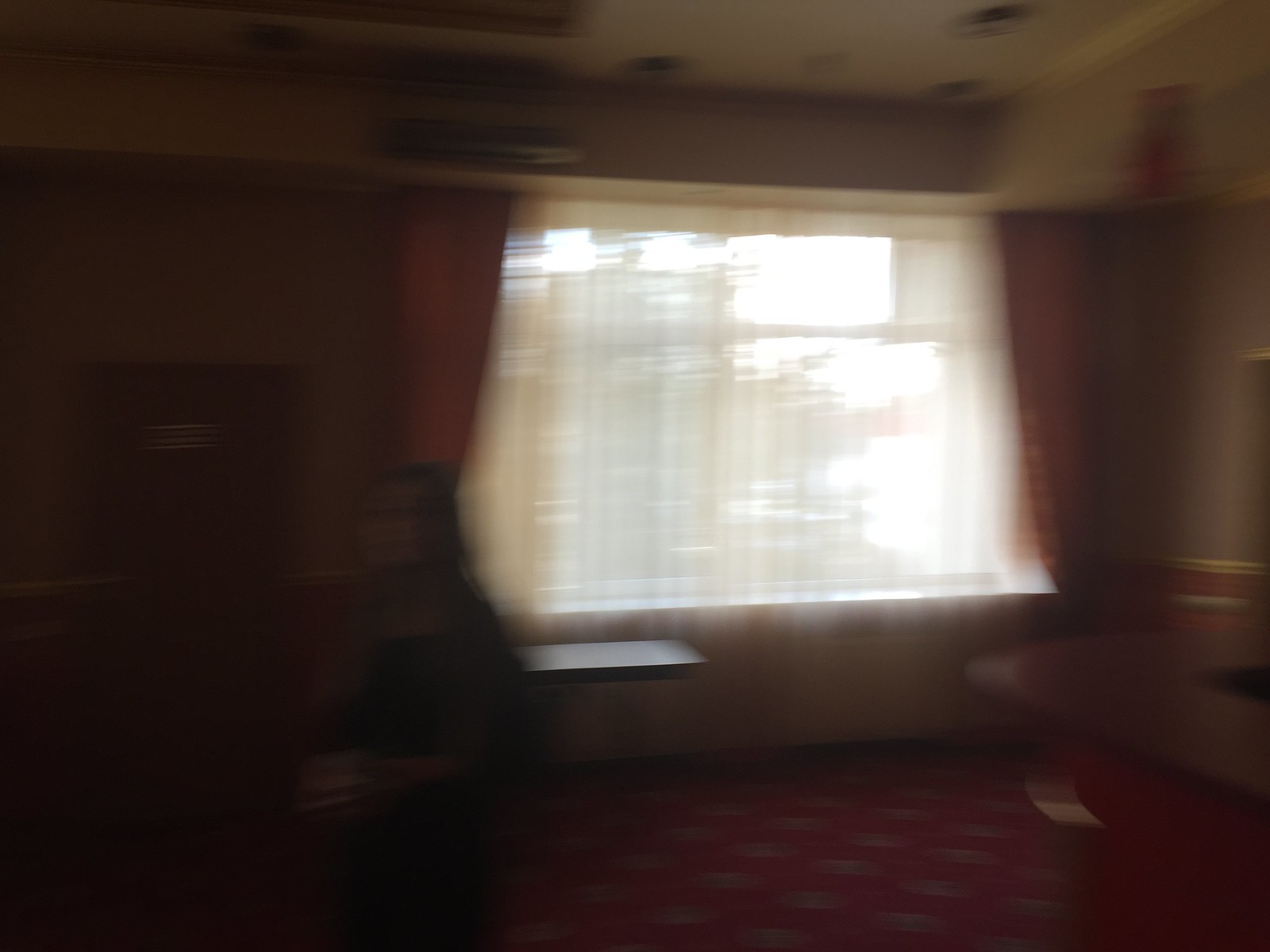This image, albeit extremely blurry, depicts a room with the viewer facing a window adorned with a delicate, transparent gauzy white curtain complemented by darker curtains on either side. At the top of the frame, a ductless air conditioning unit appears to be mounted, suggesting climate control within the space. The lower portion of the image hints at the presence of a small table, though the indistinctness and darkness obscure additional details and elements in the room.